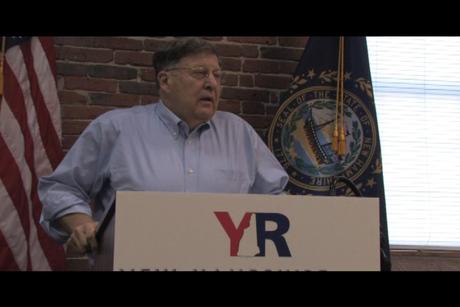This is a horizontally aligned photograph of a man, approximately in his 50s or 60s, standing at a white podium with "YR" prominently printed on the front, the 'Y' in red and the 'R' in black. The man is a white male with short brown hair on the sides and longer hair on top, combed over to his right. He's wearing glasses and a light blue button-down Oxford shirt, with sleeves rolled up, gripping the podium with his right hand while his left arm is partially obscured behind the podium. 

His facial hair features a light grey mustache, and he appears clean-shaven otherwise. Behind him, there is a red brick wall with horizontally aligned bricks. To his left, partially visible in the upper left corner, is a rumpled American flag, showing the blue field with white stars and red and white stripes in a wavy pattern. On the other side, a blue flag, possibly a state flag of New Hampshire, features a yellow state seal with elements including a sailboat surrounded by Roman numerals and a golden circle, adorned with two yellow tassels.

In the background, a faint blue PowerPoint presentation or slide projector screen can be seen to the right, displaying indistinct text and a series of horizontally aligned lines that darken towards the bottom. Overall, the setting suggests this could be a government announcement or meeting.